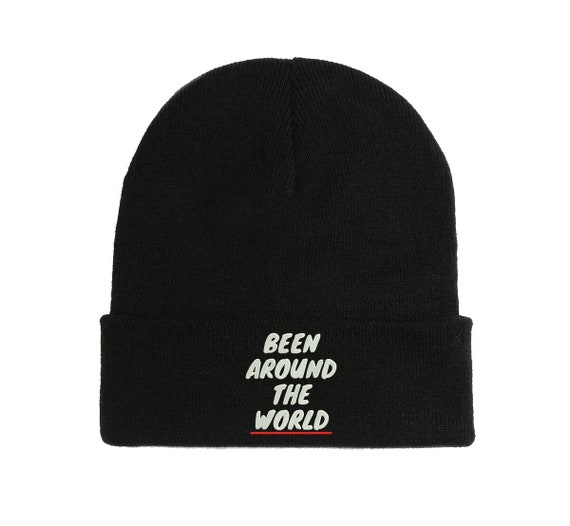The image showcases a black woollen hat, typically referred to as a beanie, scully cap, or hipster beanie, prominently centered on a white background. This close-up shot highlights the hat’s intricate knit material, with a seam creating an almost pleat-like effect at the top. The hat is folded up at the rim, which features bold, italicized white writing that reads "BEEN AROUND THE WORLD," with the word "WORLD" underlined in red. The hat lies flat, taking up nearly the entire frame of the well-lit image, and has a dome shape with no pom-pom or additional embellishments. Designed for an adult, this beanie appears warm, perfect for cold winter days.